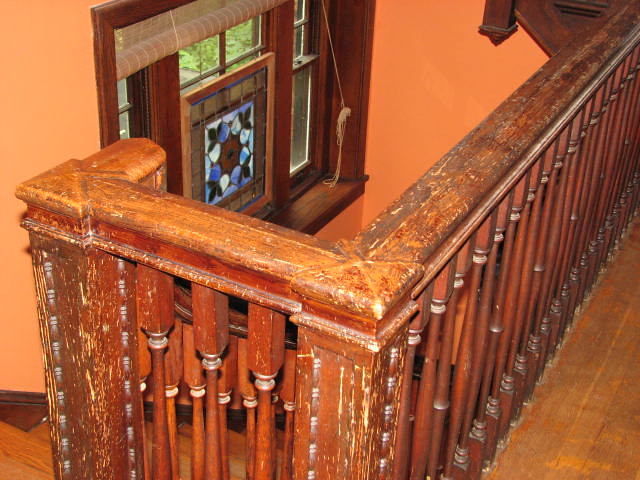The image depicts the view from the second landing of an aged wooden staircase in a vintage, historic house reminiscent of the 1920s or medieval times. The wood railings are worn and scratched, evoking a sense of antiquity. The house features intricate glass windows adorned with murals, including a notable one with a blue, white, and brown flower motif, reminiscent of old-school church windows. The walls are painted in warm hues of orange and pink, enhancing the historic atmosphere. This grand, historic home suggests a place where significant figures, perhaps even a president, might have resided.